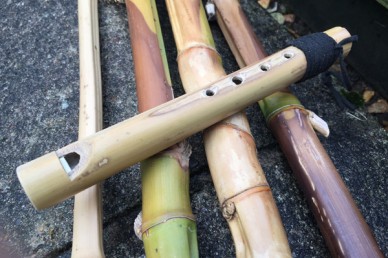The image showcases a meticulously handcrafted bamboo flute, positioned diagonally atop four evenly spaced bamboo stalks that run vertically from the top to the bottom of the frame. Each bamboo stalk exhibits a natural blend of green, brown, and tan hues. The flute itself is fashioned from freshly cut bamboo, featuring four precisely carved finger holes and an airflow notch. A black rope is tied at the end of the flute, suggesting it might be used for hanging. The scene is set against a dark granite rock background, scattered with a few yellow leaves on the right side, adding a touch of natural rustic charm.